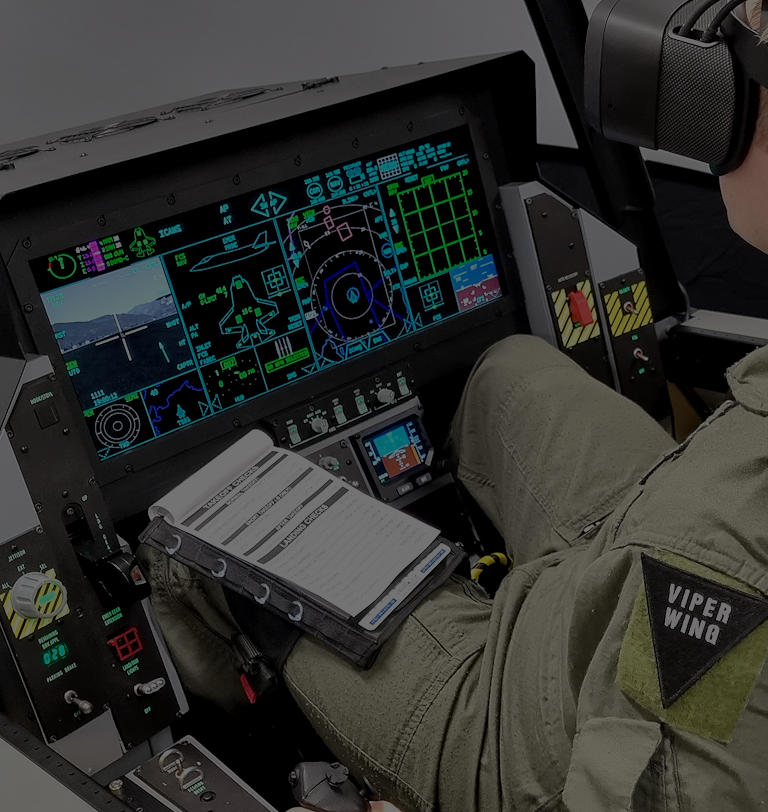The photograph is a detailed, dimly lit, square-format image showcasing the interior of a sophisticated cockpit flight simulator, capable of replicating the F-16, F-35, or F-18 fighter jets. The viewpoint is from above, looking down at an individual who is seated on the right side of the image, facing the left where a monitor with brightly colored displays can be seen. The person is deeply engaged with the simulation, wearing a black virtual reality headset, and is attired in a khaki-colored shirt and matching pants. A notable feature on their clothing is a black triangle on their shoulder with the white text "Viper Wing." In their lap rests an open notebook on their left leg, displaying a folded white notepad with several lines of text. The cockpit is replete with various controls, buttons, switches, joysticks, and an instrument panel with gauges, all contributing to the realistic feel of the simulation environment. The background is indistinct, possibly white or gray, adding to the focus on the detailed setup and the individual's immersive experience in the simulator.